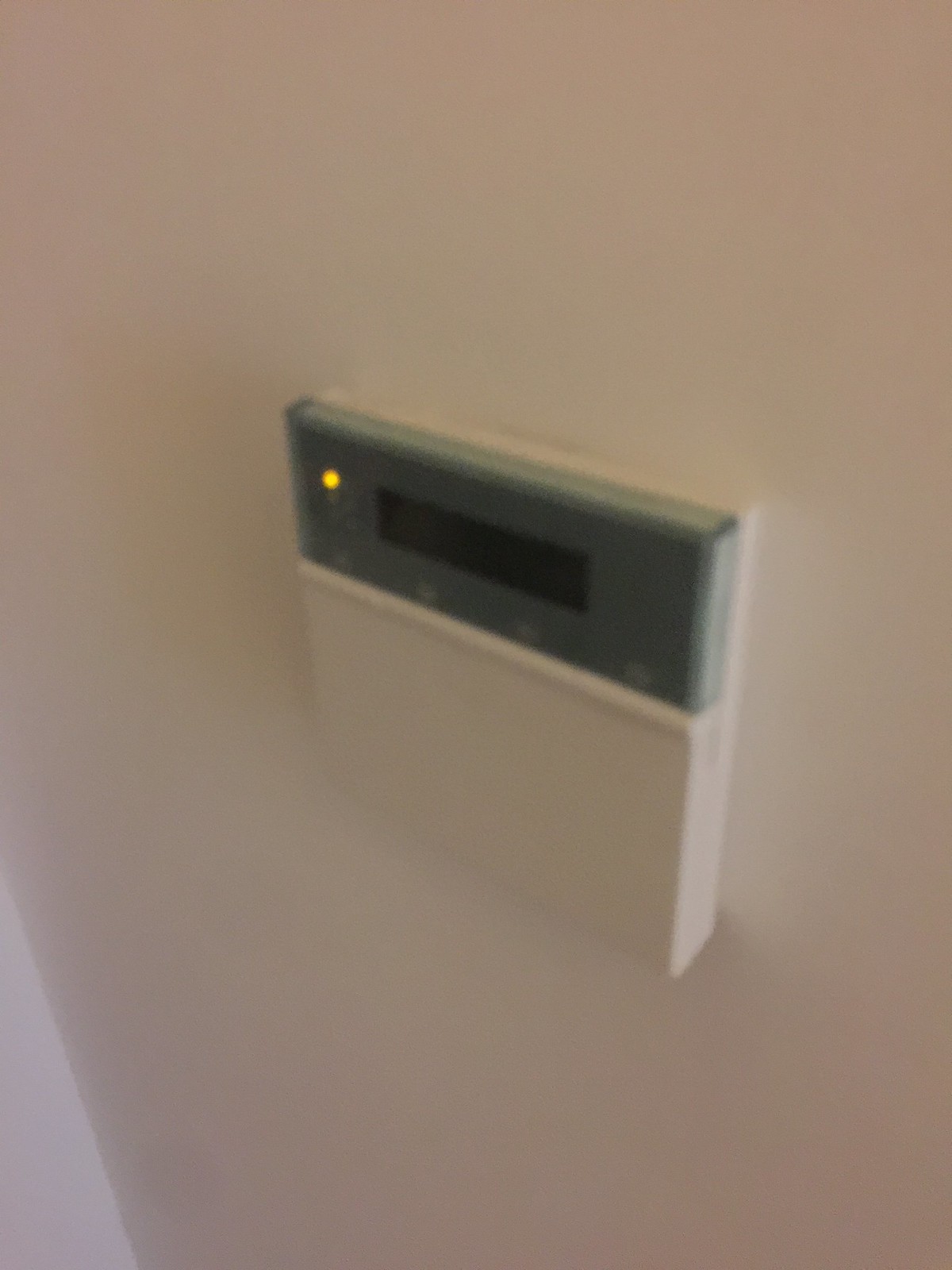A grey rectangular structure occupies the majority of the image, featuring a slight triangular section colored in a lighter shade of grey. Positioned centrally, a protruding element resembles a letterbox. This object has a dark grey top with a rectangular slot and a lighter grey lower half, suggesting it could store items. Notably, a bright yellow light is located on the left-hand side of the slot, adding an unusual detail that differentiates it from a typical letterbox and raises questions about its function. The overall design and the presence of the light give it a unique and intriguing appearance, unlike anything commonly seen before.